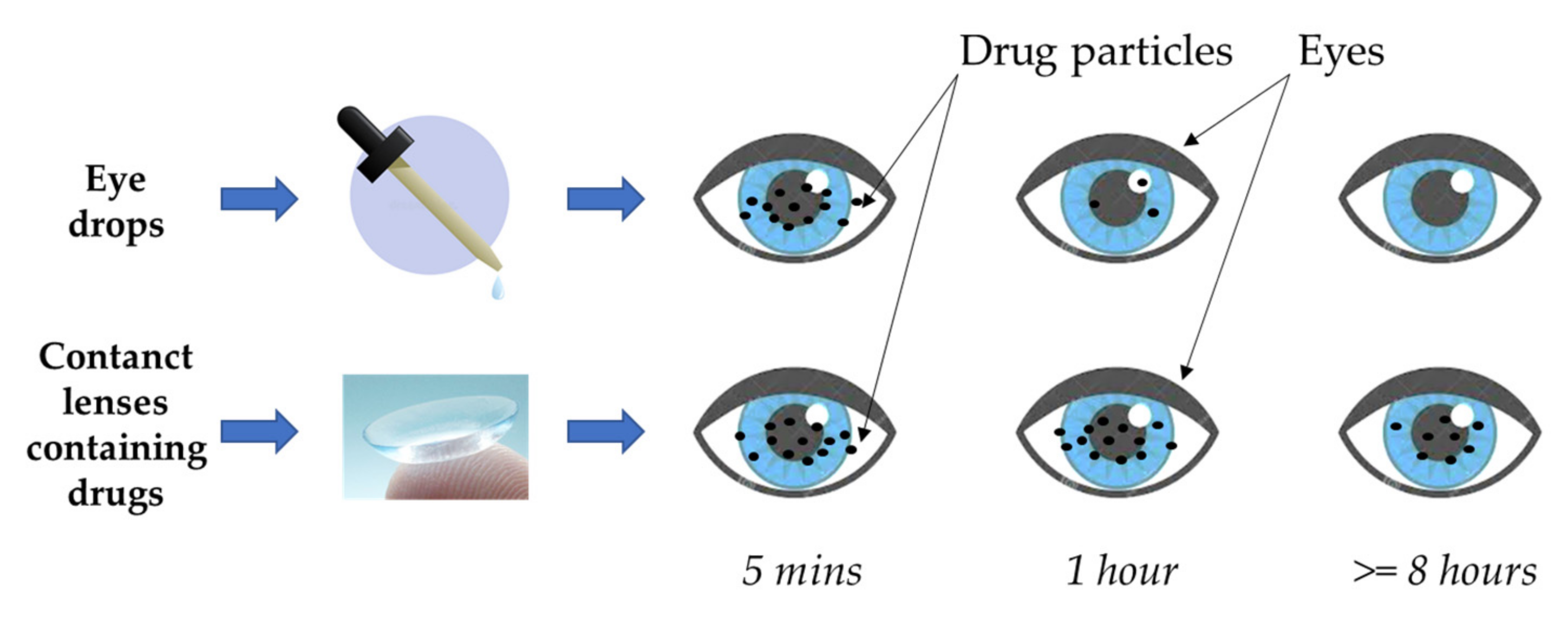The image is a comprehensive, step-by-step visual guide set against a solid white background, illustrating the effectiveness of eyedrops versus drug-infused contact lenses for eye treatment. The diagram is split into two main sections:

**Section 1: Eyedrops**
- A blue arrow guides the viewer's eye from the word "eyedrops" to an image of an eyedropper dispensing a drop.
- Another blue arrow points to an eye with black dots labeled "drug particles," showing the initial state of the eye.
- Following the blue arrow, the next image demonstrates the eye with fewer particles.
- The final image in this sequence displays a clear eye, indicating the complete effectiveness of the eyedrops.

**Section 2: Drug-Infused Contact Lenses**
- On the bottom left, the caption "contact lenses containing drugs" is accompanied by an image of such a lens.
- An arrow points to the lens placed on a finger, ready for application.
- The final part of this sequence includes images of an eye at three time intervals: labeled "5 minutes," "1 hour," and "8 hours," showing the progressive disbursement of drug particles and clearing of the eye over time.

Overall, the image emphasizes that while eyedrops clear the eye relatively quickly and effectively, drug-infused contact lenses take a longer time to achieve the same result, suggesting that eyedrops might be the preferred choice for quicker eye clarity.